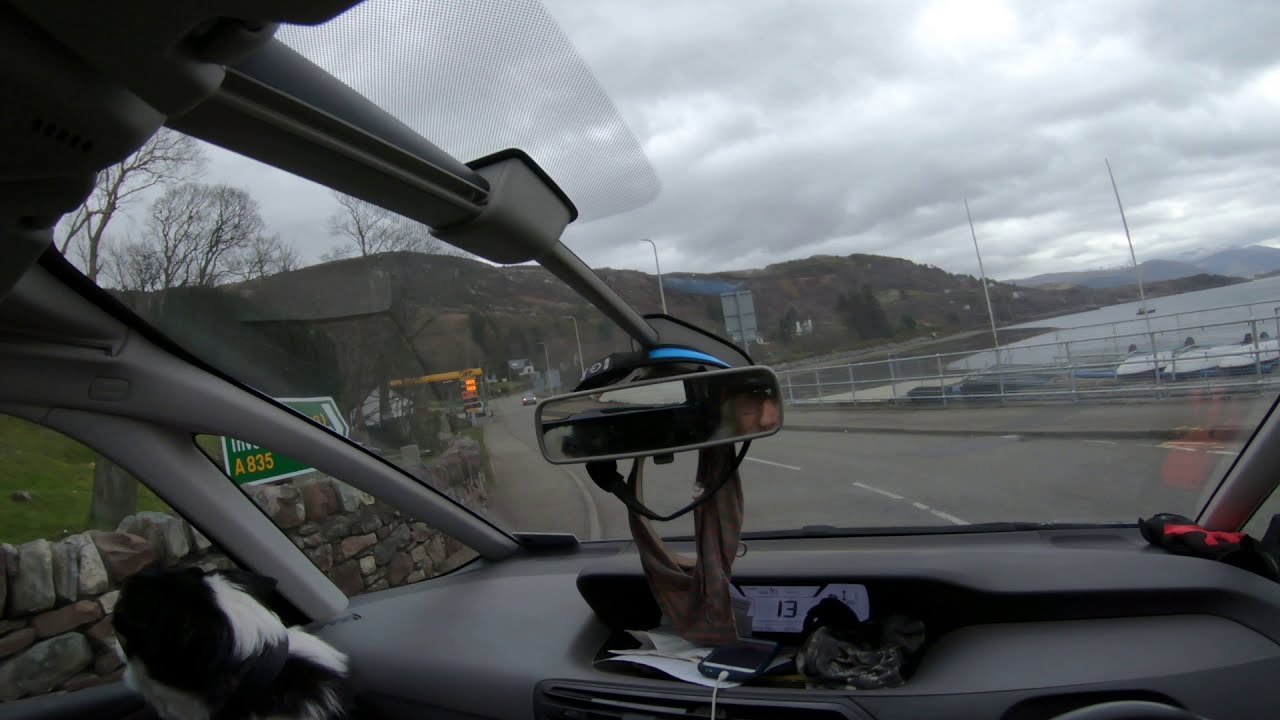This photograph, taken from inside a right-hand drive car, captures a first-person perspective through the front windshield, with the rear-view mirror prominently centered in the frame. The scene outside reveals a two-lane road flanked by scenic landscapes. On the left, hills draped in brown and green foliage rise against a backdrop of white, puffy clouds. To the right, there is a body of water, indicative of a coastal setting. In the lower left corner of the image, seated in the passenger seat, a small, black and white fluffy dog gazes out the window. The road follows the left side of the frame, hinting at the vehicle's motion through what seems to be a picturesque coastal town. Additionally, street signs, including one marked "A835," and a gas station are visible, along with some distant buildings and hills, completing the roadside vista. Inside the car, various objects, including a phone, are also seen. The overall scene conveys a serene drive through a quaint, possibly British, coastal area.